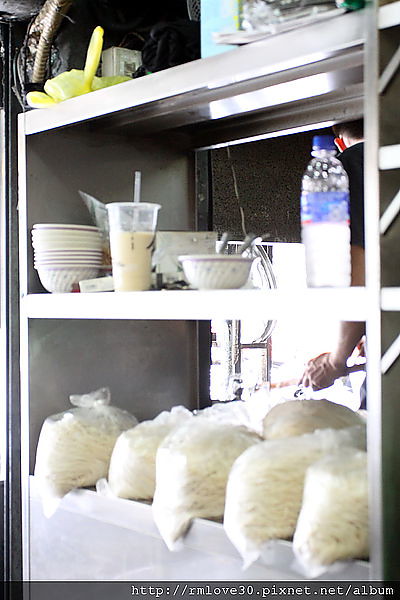This photo showcases a stainless steel shelving unit located in what appears to be a kitchen space, potentially part of a busy culinary environment. The background is dark, possibly black, and there may be a TV set behind the shelf. The top shelf is well-organized with a stack of small plastic bowls. Adjacent to the bowls is a partially consumed cup of what seems to be milk tea, placed in a plastic drink container holder. Nearby, there is another small bowl with a yellow spoon inside it. At the right edge of this top shelf, a clear plastic water bottle with a blue stripe and polka dots halfway up its length can be seen. Just above, a small flag decorates the top of the bottle. Additionally, a yellow glove might be on this shelf, suggesting that someone is working nearby. On the second shelf below, large plastic bags filled with white noodles, described as doughy and ripply, are arranged. Decorative white bowls, featuring a blue stripe and floral designs around the edges, are also evident. This image appears to be set in a bustling kitchen area, possibly hinting at ongoing food preparation and storage activities. A website address, http://rmlove30.pixnet.net/album, is visible at the bottom right, suggesting the origin or collection of this photo.